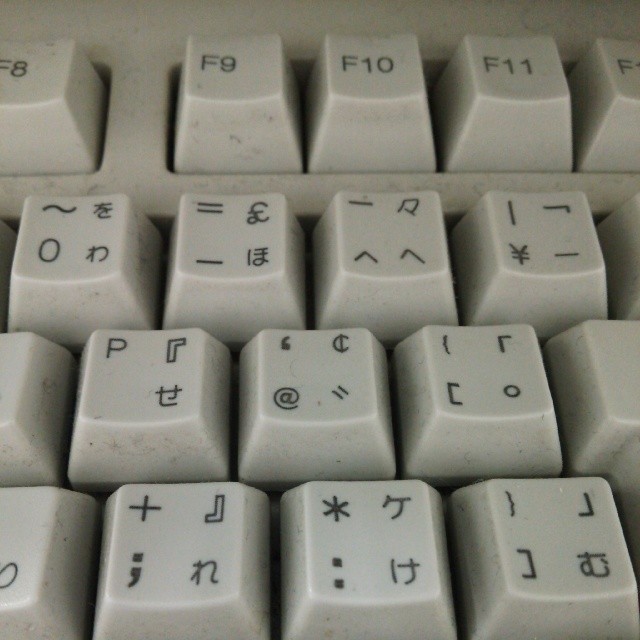This colour photograph, set in a square orientation, presents a close-up view of a computer keyboard captured from a 45-degree angle, as if looking down at it while seated. The keyboard displays an off-white, beige-cream colour, marred by visible black fluff fibers wedged between the keys. The keys themselves feature a mix of Japanese characters and English symbols, indicative of a non-English keyboard layout. Distinctly visible are keys labeled with O, P, a pound sign (£), and a yen sign (¥). The image's tight crop reveals the top left corner with partially visible function keys – from F8 to F11, and a fragment of the F12 key. Overall, the keyboard appears dusty and dirty, accentuated by darker particles dotting the keys and surrounding board.